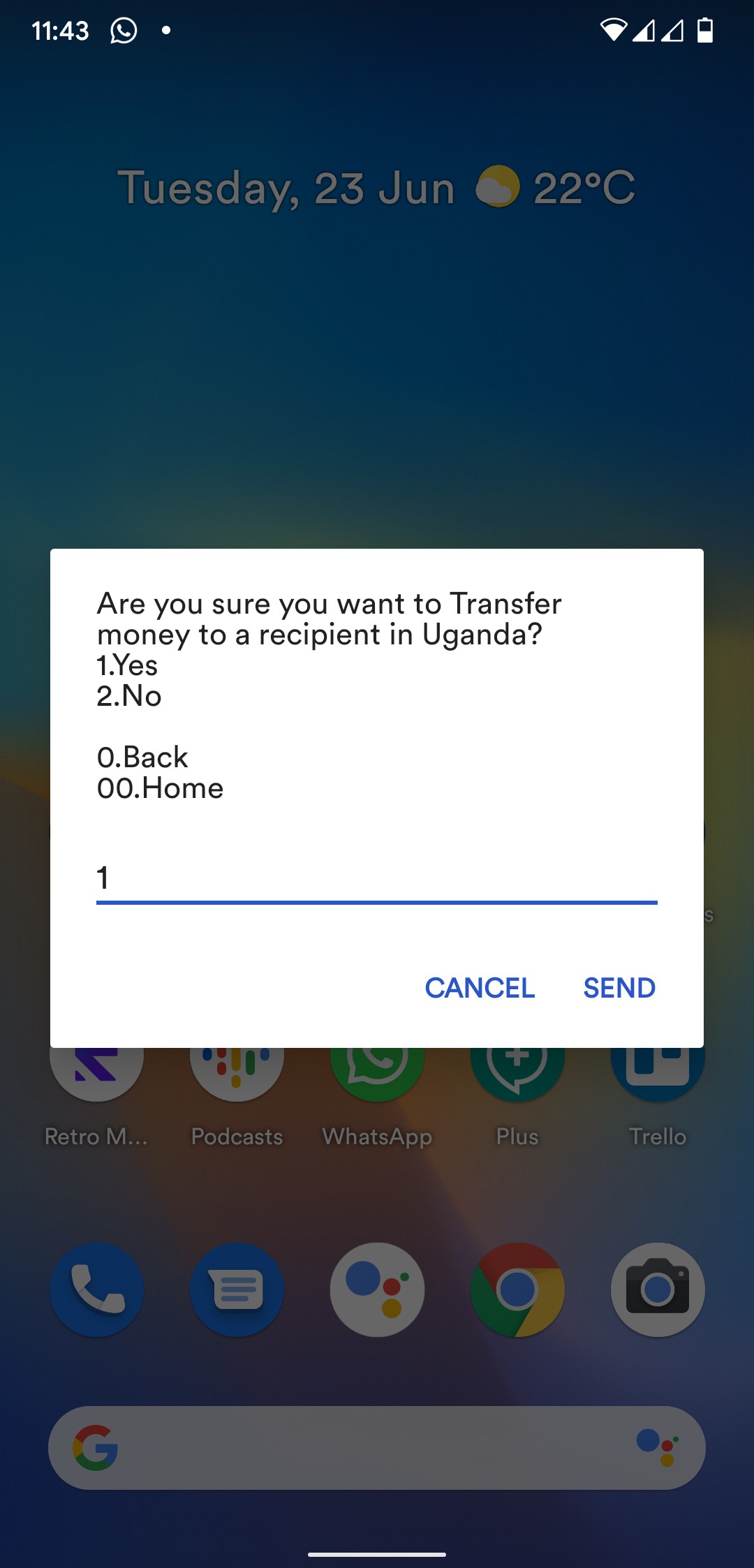A detailed caption for the image could be:

"A screenshot of a mobile device displaying various interface elements and applications. In the upper left corner, the time is shown as 11:43, accompanied by the WhatsApp icon on the status bar. The top right corner includes icons for WiFi connectivity, network signal strength indicators for SIM 1 and SIM 2, and the battery level. The date displayed is Tuesday, 23rd of June, with the weather indicating a chilly 2 degrees Celsius. A prominent dialog box in the center of the screen asks for confirmation with the message: 'Are you sure you want to transfer money to a resident in Uganda?' with options to select 'Yes' or 'No.' The home screen features various apps including Retro, Podcast, WhatsApp, Plus, Trello, Phone, Messages, Google Assistant, Google Chrome, and Camera. At the bottom, there's a Google search widget alongside the App Store icon."